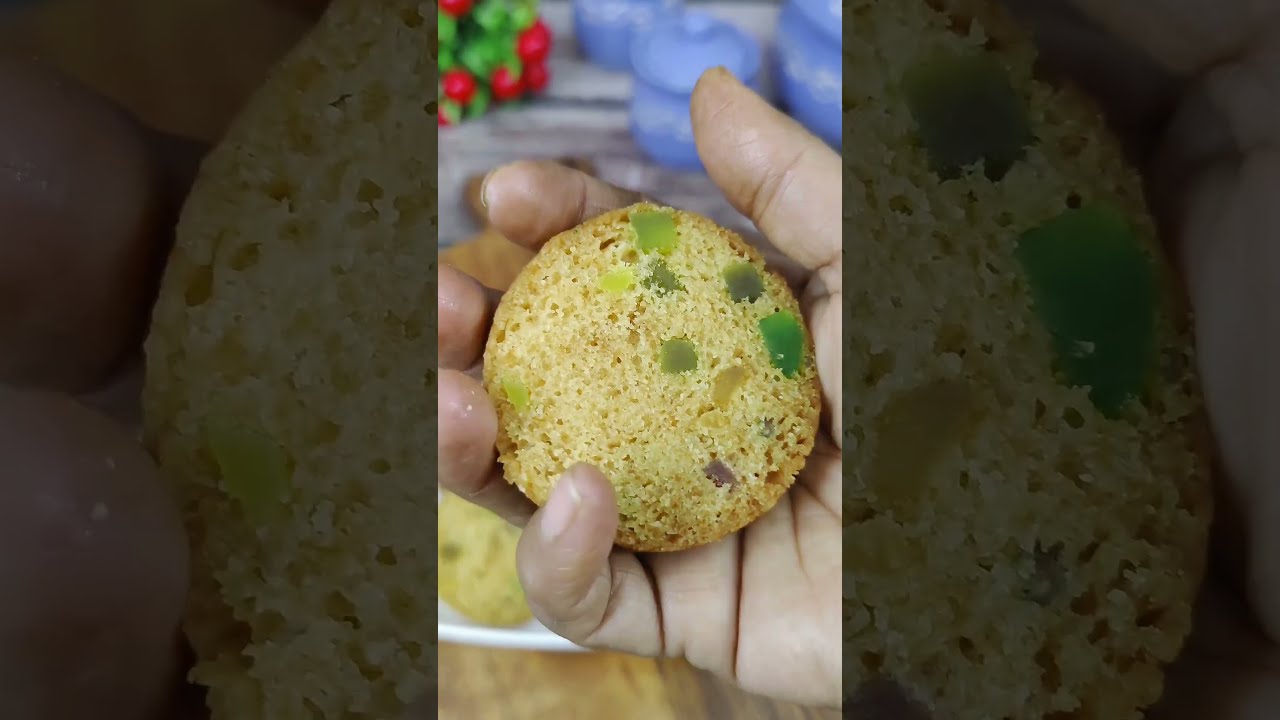In the foreground of this image, a slightly dirty hand with visible fingernails is holding a circular, sponge-like food item with green and red spots, possibly resembling candied fruit embedded within. The object appears to be yellowish and may be a slice of fruitcake or a similar baked good, with little green pieces that could be peppers or candied fruit. The background is a blurred, faded version of the same image, offering a closer view of the hand and the object. On the right side of this background, there appear to be some water jugs, while the left side includes what looks like cherry tomatoes or berries with green leaves. At the bottom of the image, a wooden floor is partially visible.